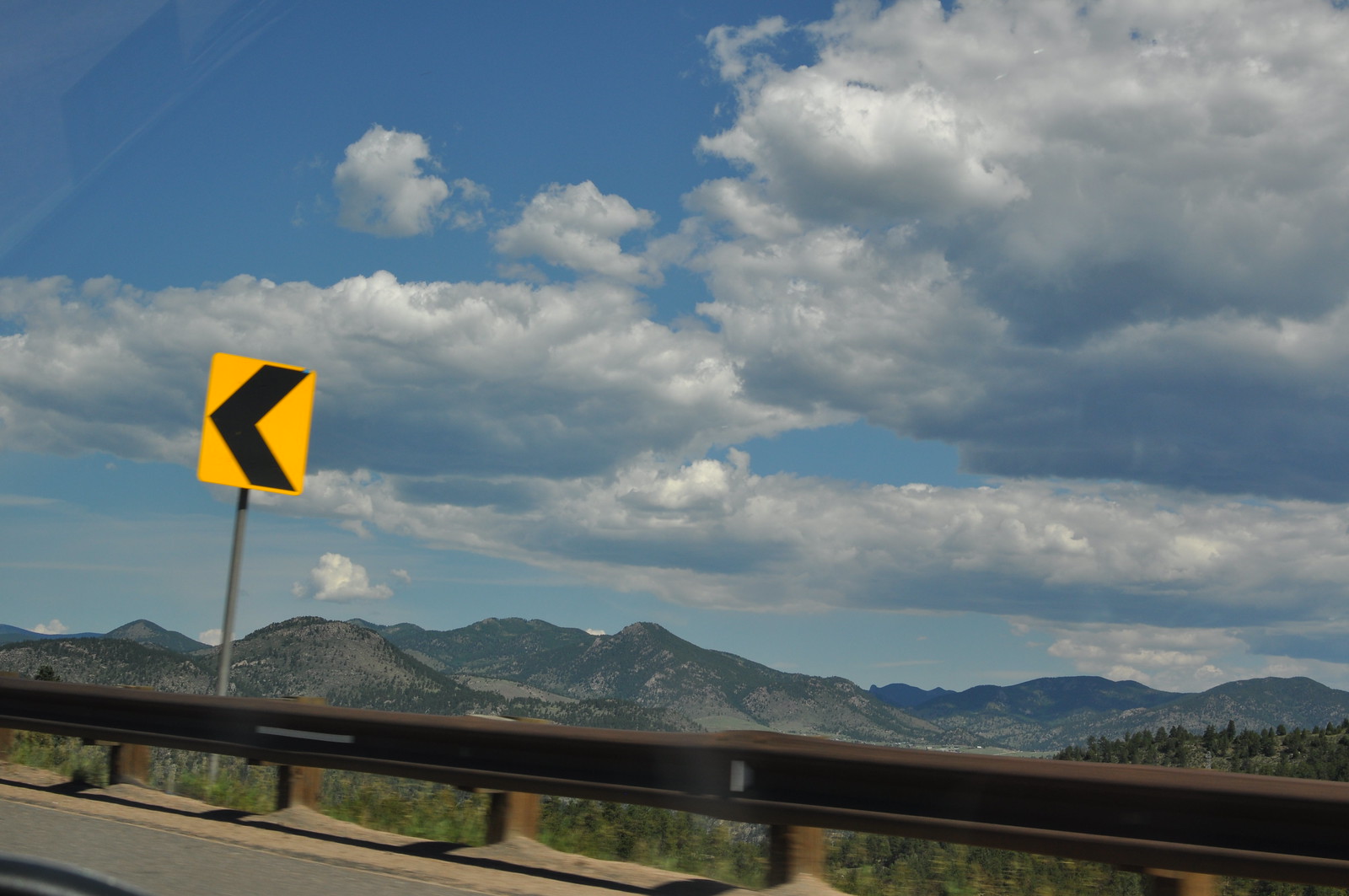The photo, taken from the passenger side of a moving vehicle, captures a picturesque scene of a sprawling mountain range in the background that stretches from the left side of the image to the right. The deep blue sky overhead is adorned with large, fluffy white clouds, some tinged with gray. In the foreground, there is a sturdy, rusted dark brown guardrail supported by wooden poles, surrounded by dirt and gravel. To the bottom right, the tops of green trees crown a hillside, hinting at a spring or summer setting. The asphalt of the road peeks through in the bottom left corner, where a yellow square road sign with a black left-pointing arrow warns of an upcoming curve.